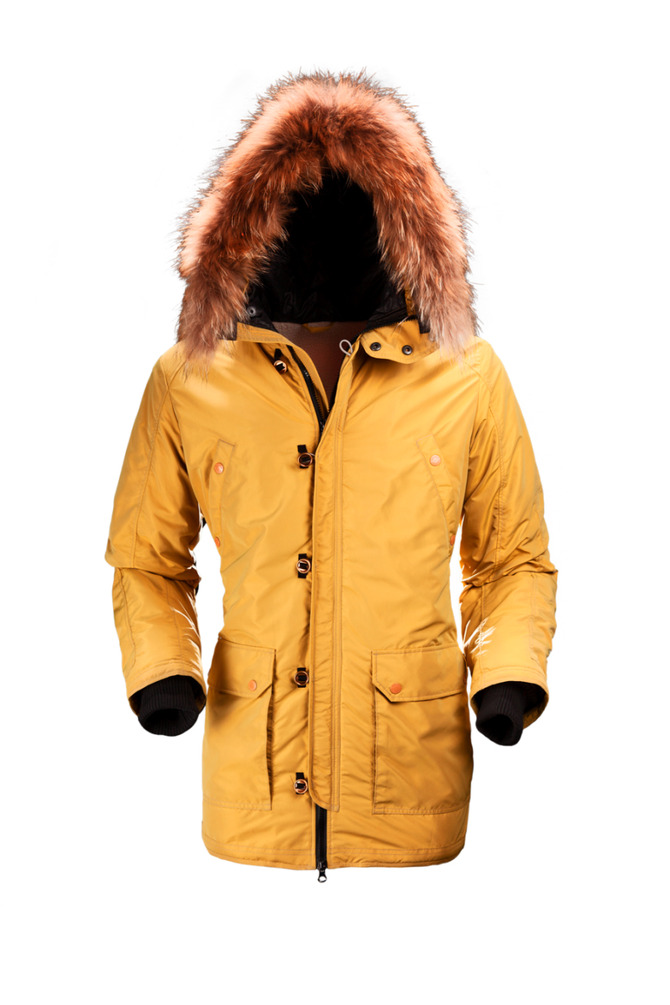This photograph showcases an empty yellow winter coat positioned as if worn by an invisible person, against a seamless white background. The coat, resembling the exact shade of a school bus with orange undertones, is long and extends down to almost the hip. The standout feature is its brown fur-lined hood, which adds a touch of coziness. The front of the coat is adorned with black metal snaps and a black zipper, complemented by the inner black lining, visible at the cuffs where the sleeves bend naturally at the elbows, emulating a human posture. Additionally, the coat features two large, practical pockets near the bottom, each secured with distinctive orange buttons, and a small yellow tag-like detail near the zipper. The realistic arrangement of the coat, despite the absence of a wearer or hanger, creates a striking, ghostly effect.